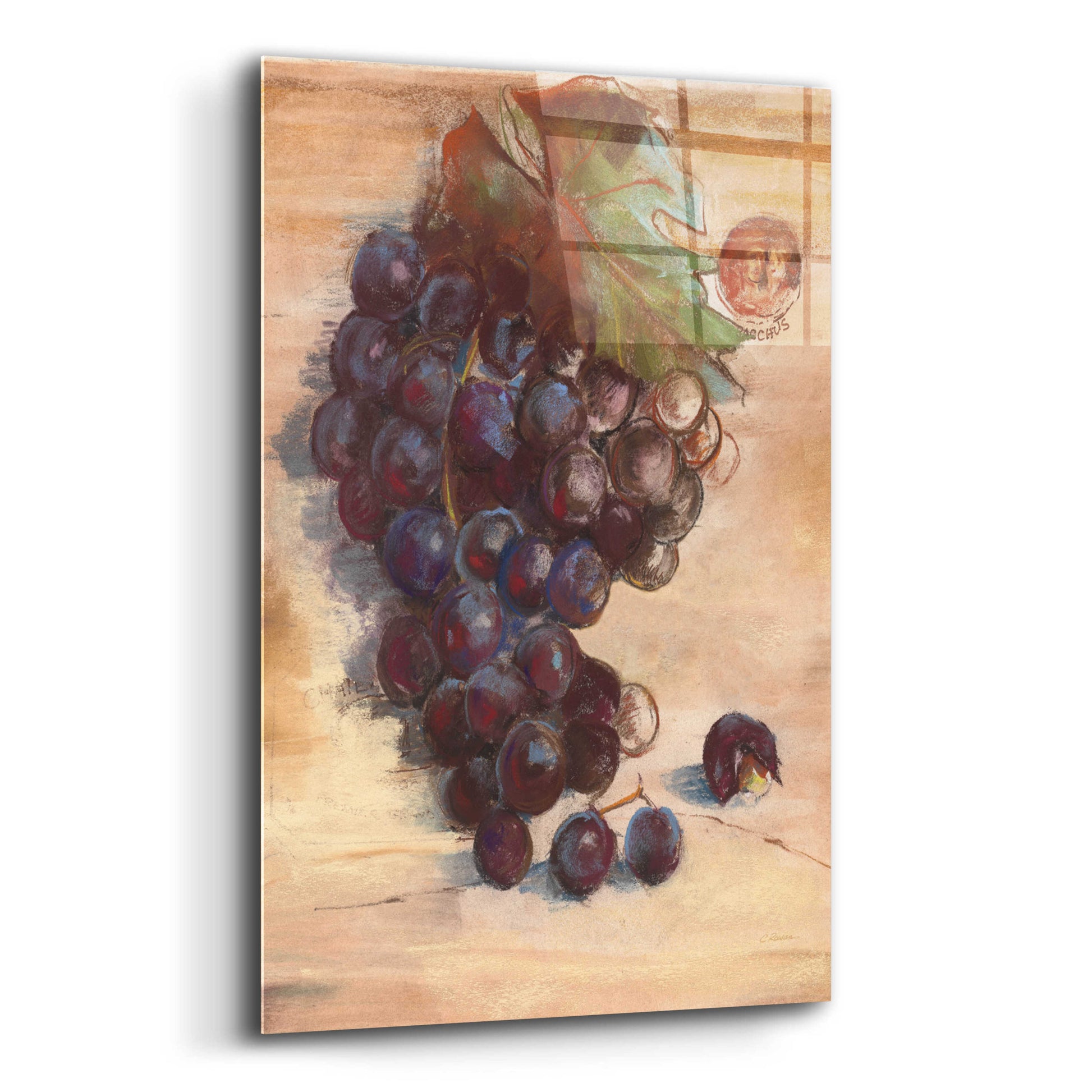The image depicts an artistic rendering of a bountiful cluster of dark red or purple grapes hanging from a leafy green vine, centered prominently on a canvas. The background of the painting is a streaky blend of beige, light brown, and tan hues, reminiscent of clay or dried ground, possibly even wood. This background gives an earthy, rustic feel, ideal for an old Italian kitchen aesthetic. In the top right corner, there is an intriguing detail—what appears to be the light shining through a window, casting shadows on the wall, and the suggestion of someone possibly looking out. This adds a layer of depth and ambiguity to the piece. A single grape has fallen and rests on the lower right side, appearing burst open, adding a touch of realism to the scene. The artist has skillfully captured the juiciness and vitality of the grapes, which are rendered in such vivid colors and detail that they seem almost tactile. There is also a jagged green leaf at the top of the cluster, with some faintly visible letters or label markings, further adding to the painting's complexity and allure. The overall composition is bright, colorful, and evocative, making it a charming and picturesque piece suitable for kitchen decor.